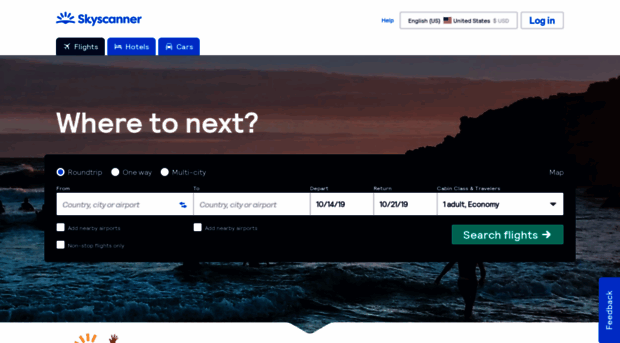The screenshot depicts a Skyscanner web page with a predominantly white, blue, dark blue, and green color scheme. At the top left, the site’s logo, "Skyscanner," is displayed in blue font accompanied by a graphic of a sun rising over the horizon, also in blue. Adjacent to the logo is a blue hyperlink labeled "Help," and to its right, there is a language setting "English (U.S.)" alongside an American flag icon. The currency is set to U.S. dollars. 

Further to the right, there is a white, rectangular "Login" button with blue text. Below this main navigation bar is a dark blue tab labeled "Flights" featuring an airplane icon. Adjacent to it are two tabs in lighter blue - one for "Hotels" with a bed icon and another for "Cars" with a vehicle icon.

Dominating the main section of the page is a background image of a sunset beach overlaid with the text "Where to Next?" in white font. A pop-up form sits centrally, designed for booking flights. It offers options for round-trip, one-way, and multi-city travel, with "One-way" currently selected. Input fields are available for the departure and destination locations, as well as for setting travel dates showing "Departure: 10-14-19" and "Returning: 10-21-19." The form indicates one adult traveling in economy class, and at the bottom of the form is a prominent green "Search Flights" button.